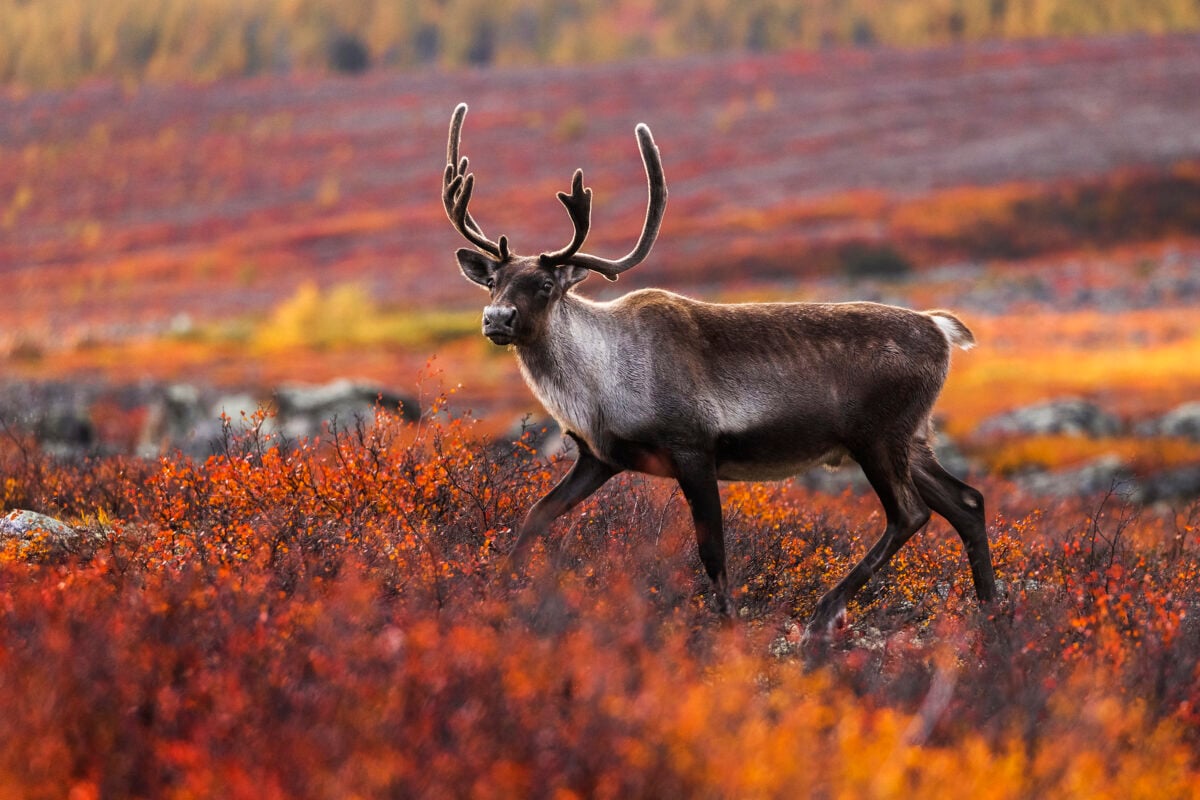In the center of the photograph, a juvenile reindeer is captured in mid-stride, walking towards the left. The reindeer is adorned with velvet antlers and has a brown and white fur coat, with its brown covering most of its body and its white fur accentuating its neck and tail area. The animal looks towards the camera, slightly to the left, showcasing its black nose and intricate antlers. The reindeer stands on a vibrant fall field filled with small shrubs and tall grass, dyed in shades of red, orange, pink, and yellow. The background is out of focus, subtly revealing blurred trees and rocks, emphasizing the picturesque autumnal setting during the daytime.